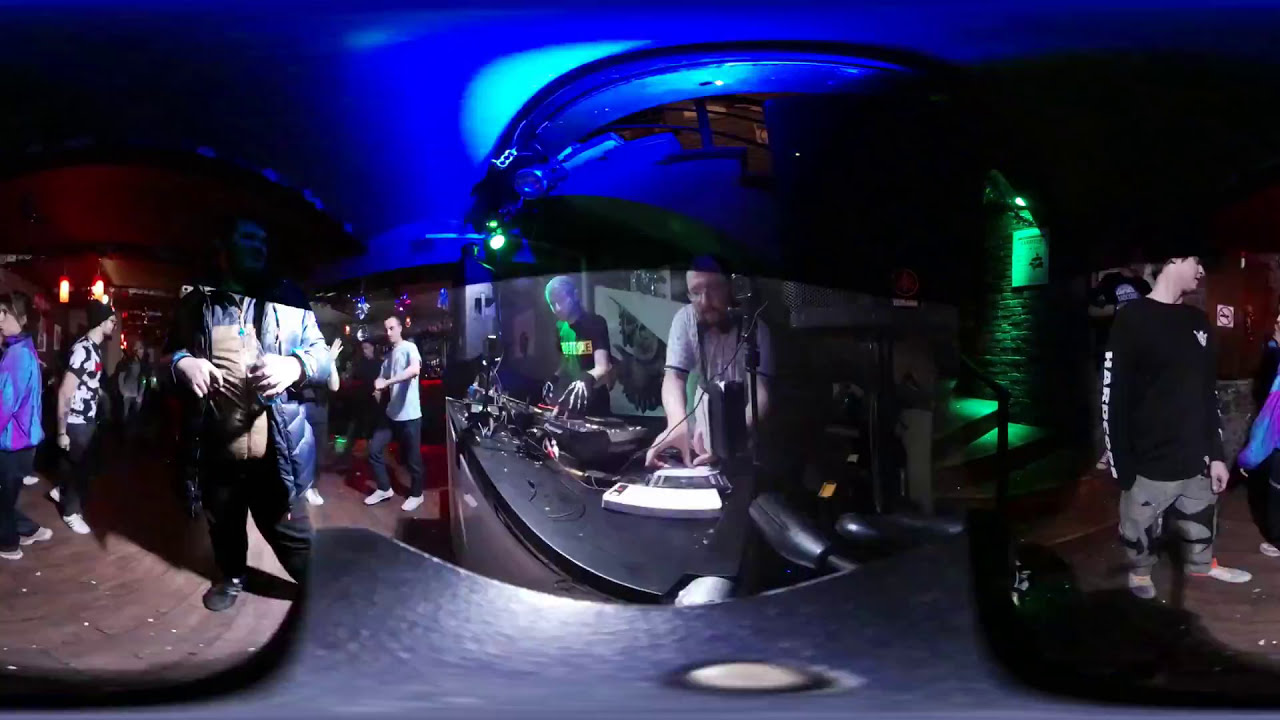The image captures a vibrant and bustling club scene, featuring a dance floor and a DJ booth prominently positioned in the center. The DJs, integral to the lively atmosphere, are equipped with various music equipment and both wear headphones; one wears a white short-sleeved shirt, while the other sports a black shirt with a yellow image emblazoned on it. Ambient lighting in hues of blue, green, purple, gray, black, white, yellow, and red illuminates the scene, with a noticeable blue light reflecting throughout the ceiling and over the top of the DJ equipment. Surrounding the DJs, groups of people are seen dancing and socializing. To the right, one person stands apart from the dance floor, while others on the left seem to enjoy the music and revel in the club's lively energy. The setting, a dark indoor environment, possibly also serves as a bar given the orange lights in the background and the wood flooring underfoot. The layout suggests the photograph might be a 360-degree panoramic view, adding to the chaotic but immersive experience of the scene, with an age group appearing to be mostly between 25 and 35 years old. The DJs are located under a staircase that is illuminated, with blue lights adorning the top and green lighting the bottom, adding to the overall dynamic and festive atmosphere.